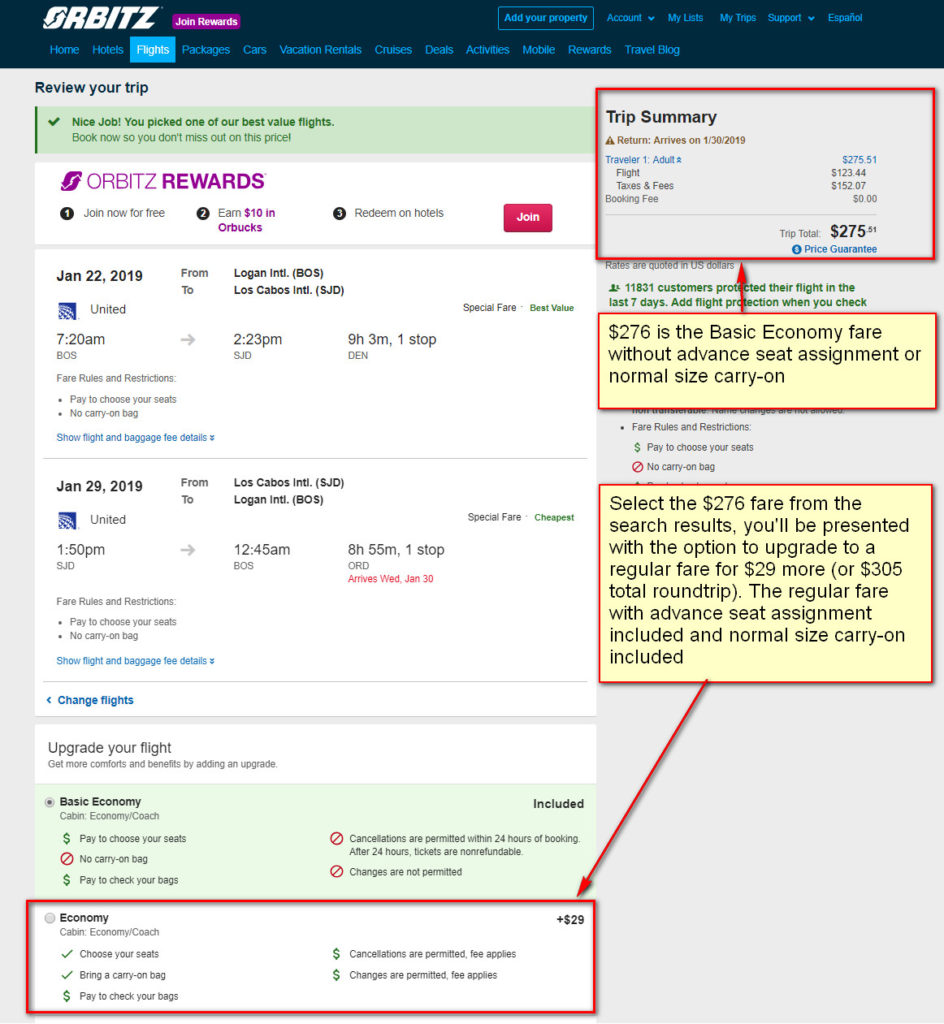This is a detailed screenshot of the Orbitz website, showcasing several flight itineraries. At the top of the image, a dark blue navigation bar spans across the page. On the top left, the slanted text logo "Orbitz" is displayed prominently. To the right of the logo, a purple button labeled "Join Rewards" is visible. Further right along the same row are six options: "Add to Property Account" (a drop-down menu), "My Lots," "My Trips," "Support" (another drop-down menu), and "Español."

Below this dark blue bar, a secondary navigation menu is present, also within a blue section. It lists several clickable options: "Home," "Hotels," "Flights" (which is highlighted in blue, indicating the current page), "Packages," "Cars," "Vacation Rentals," "Cruises," "Deals," "Activities," "Mobile Rewards," and "Travel Blog."

Just beneath the navigation bars, the section titled "Review Your Trip" is visible, displaying a detailed flight itinerary. The itinerary includes various sections that are highlighted in red boxes for emphasis.